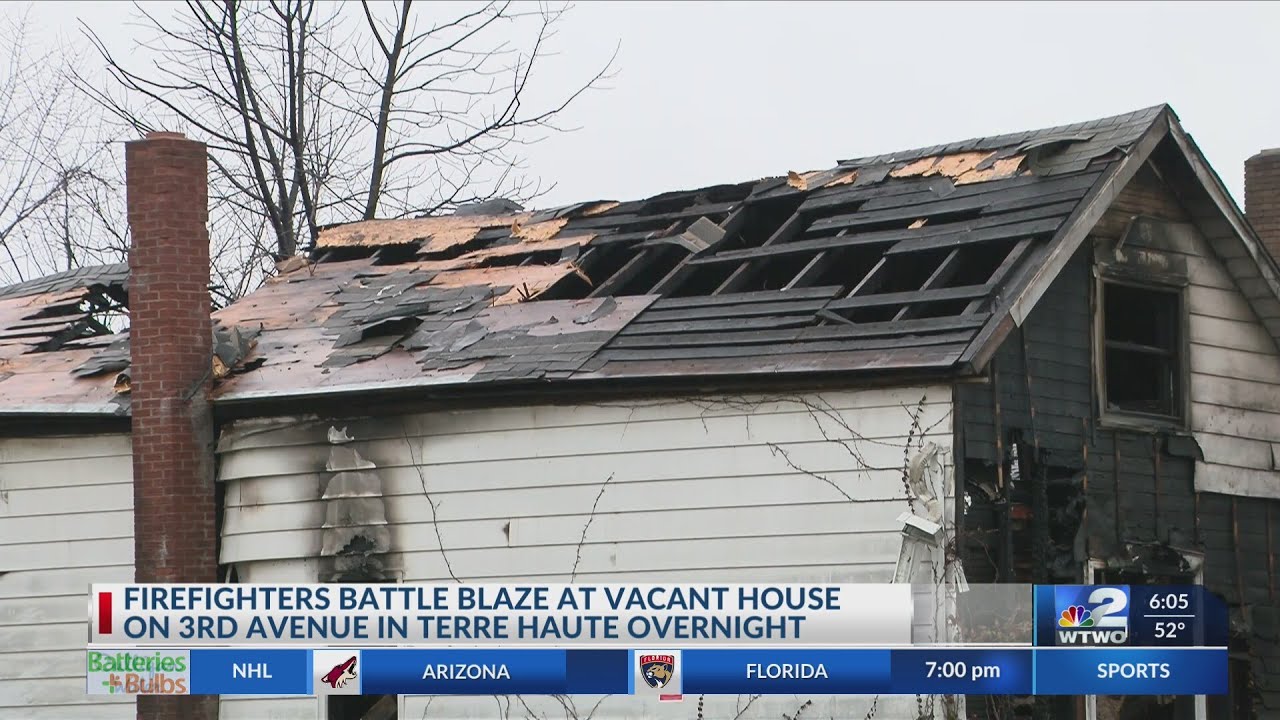This detailed caption is meant to encapsulate the shared and repeated elements from all three descriptions, providing a comprehensive overview of the scene:

"A photograph from a news broadcast depicting a severely burnt and partially collapsed house with white wooden paneling. The house features a red brick chimney on the left side, which exhibits some smoke damage. Most of the roof is destroyed, reduced to charred rafters with large sections missing. The front and side of the house are marked by heavy fire and smoke damage. A dark-outlined window is centrally located on the front side, surrounded by grey-tinged panels. Behind the house, leafless grey trees stand against an even grey sky. The newscast chyron at the bottom of the screen relays the headline: 'Firefighters battle blaze at vacant house on 3rd Avenue in Terre Haute overnight,' alongside various graphics. On the left, there's a blue diagram featuring a green and orange 'Batteries Plus Bulbs' logo, followed by 'NHL,' 'Arizona' with a cartoon fox logo, 'Florida' with an emblem of a bobcat, '7pm,' and 'Sports.' To the right, the NBC peacock logo with '2WTWO' is displayed, alongside '605, 52 degrees.'"